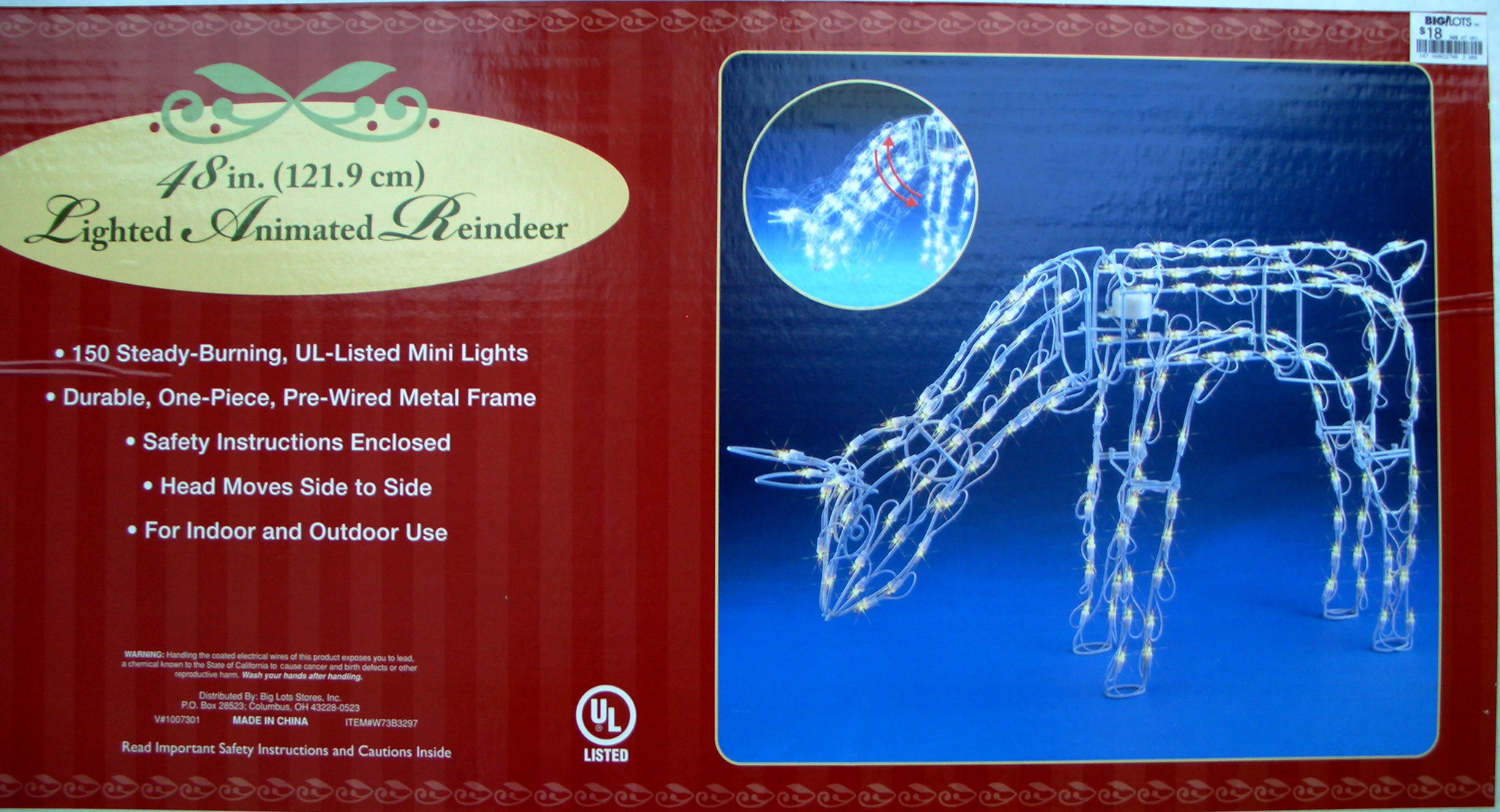The image appears to be a highly detailed promotional poster for a festive holiday product, specifically a decorative, animated reindeer. The background of the poster is a deep red, creating a striking contrast with other elements. On the top left, there is an oval-shaped, yellow-beige section that prominently displays "48-inch (121.9 cm) lighted animated reindeer" in green lettering. The reindeer, crafted from a durable, one-piece pre-wired metal frame, is adorned with 150 steady burning UL-listed mini-lights, which emit a bright white glow. The reindeer's head is animated, designed to move side to side, enhancing its lifelike appearance. This section also emphasizes its versatility for both indoor and outdoor use, with safety instructions included for proper setup.

Below this description, five detailed call-outs provide further features: the first highlights the 150 mini-lights, the second underscores the durable metal frame, the third assures the presence of enclosed safety instructions, the fourth mentions the head movement, and the last reiterates its suitability for various settings.

On the right side of the poster, a blue square showcases the reindeer in action, bathed in yellow light bulbs, against a dark background. This visual complements the left-side text, completing the promotional message with a comprehensive view of the festive decoration in a real-world setting.